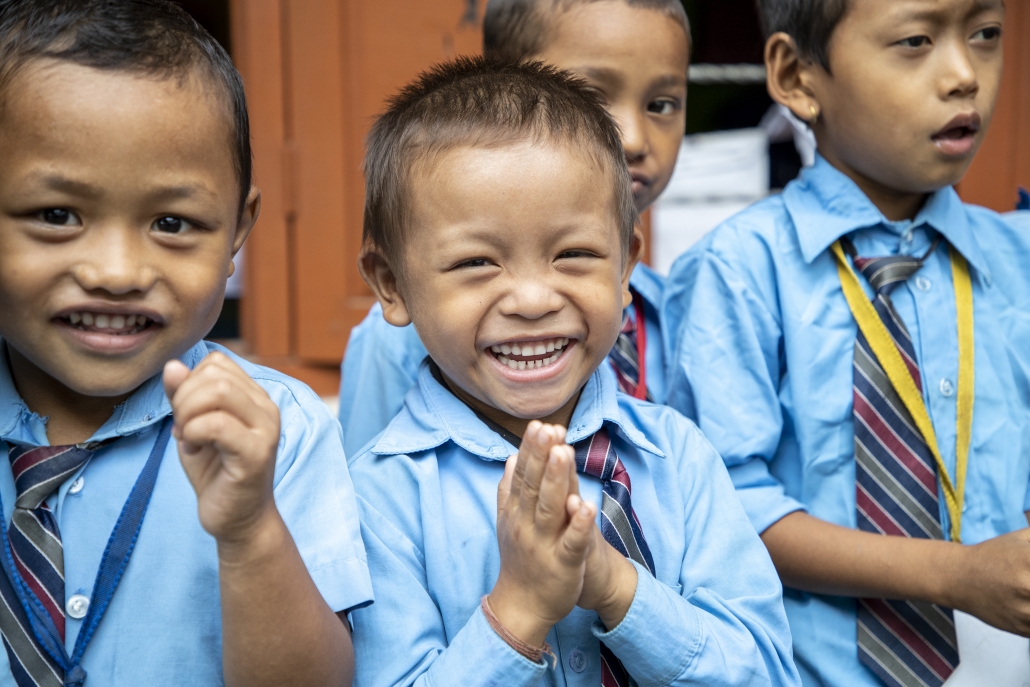The image features four young boys, seemingly of diverse backgrounds with dark skin tones, dressed in coordinating blue dress shirts and striped neckties in shades of blue, burgundy, and gray, accented by thin white stripes. Each boy displays short hair, embodying a neatly groomed appearance. Notably, one boy, standing second from the left, is clasping his hands together in a gesture reminiscent of praying while smiling brightly. His immediate neighbor to his left raises a left fist triumphantly, also beaming at the camera. On the right, one boy gazes directly into the lens of the camera with a composed expression, while the boy farthest to the right stands out with his mouth open in apparent surprise, an earring gleaming on his right ear.

In the background, a light brown building with distinct openings, possibly doors, and windows, provides a subtle setting for the boys’ lively interactions. Observers can also spot varied colorful cords draped around the boys’ necks—one in yellow, one in red, and one in blue—with one boy notably lacking a visible cord. Wooden cabinets seen at the sides hint at an indoor environment, possibly a school or community center, contributing to the photograph's warm and orderly atmosphere. The overall scene captures a moment of shared joy and camaraderie among the boys, suggesting a special event or typical school day where they are evidently happy and engaged.